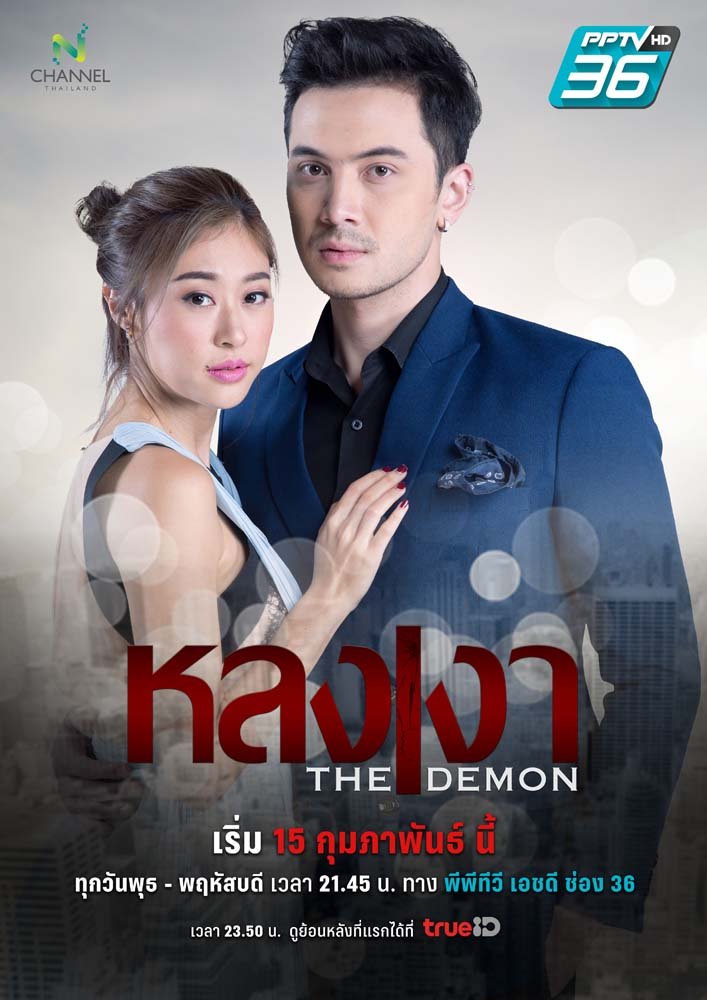The image appears to be a poster for a Thai TV show, prominently displaying the title "The Demon" in English. The top left corner features the words "Channel" and "Thailand" in dark gray font, while the top right corner has a black box with "HD" in white and the number "36" beneath it. To the right of "Channel Thailand," a teal box with "PPTV" in white font is visible. The poster has two main figures: a man and a woman. The man is dressed in a blue suit with a black collared undershirt, and a silk scarf peeks out of his pocket. He’s posed to the right of the woman, who has her hair in a loose bun with side bangs and appears to be wearing a sleeveless blue outfit, possibly overalls, over a black top. Both appear to be of Asian descent. The background includes a ghostly image of a city towards the bottom, along with various text in Thai written in white, red, and blue. There is an English phrase "the demon" prominently featured among the Thai characters. At the very bottom, "true ID" can be seen alongside part of a date that reads "2350," reinforcing the idea that this is a promotional poster, likely for a TV channel or streaming service.